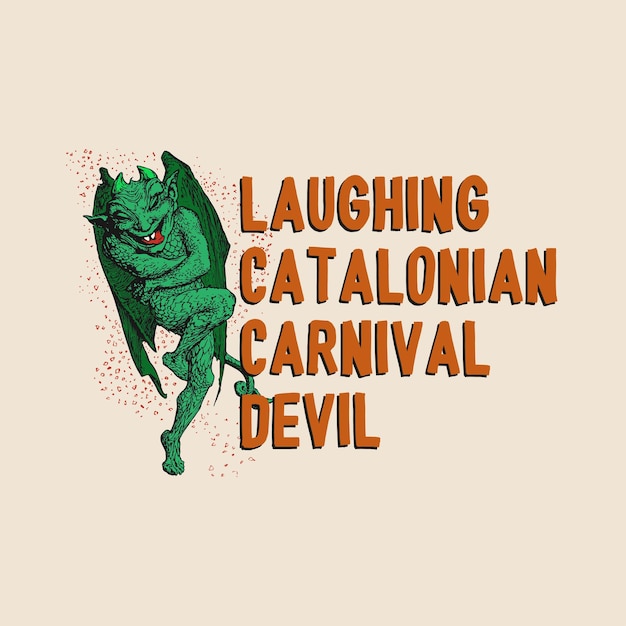The square image, measuring five inches on each side, features a light beige background with an orangish tinge. Centrally aligned are four large lines of dark orange text with thin black shadows reading "Laughing Catalonian Carnival Devil." To the left of the text stands a whimsical green devil character. This devil, adorned with green wings, horns, and pointed ears, stands on his left leg with his right leg bent at the knee, so his right foot hides behind his left knee. His curled, green tail extends towards the "C" and "D" in "Carnival" and "Devil." 

His arms are crossed in front of his green-scaled torso, contributing to a mischievous stance. He laughs with his mouth wide open, showcasing a red tongue and two sharp upper fangs, while his closed eyes suggest he's reveling in joy. His large wings are folded close to his body, and he is surrounded by orange circles resembling confetti, adding to the festive atmosphere.